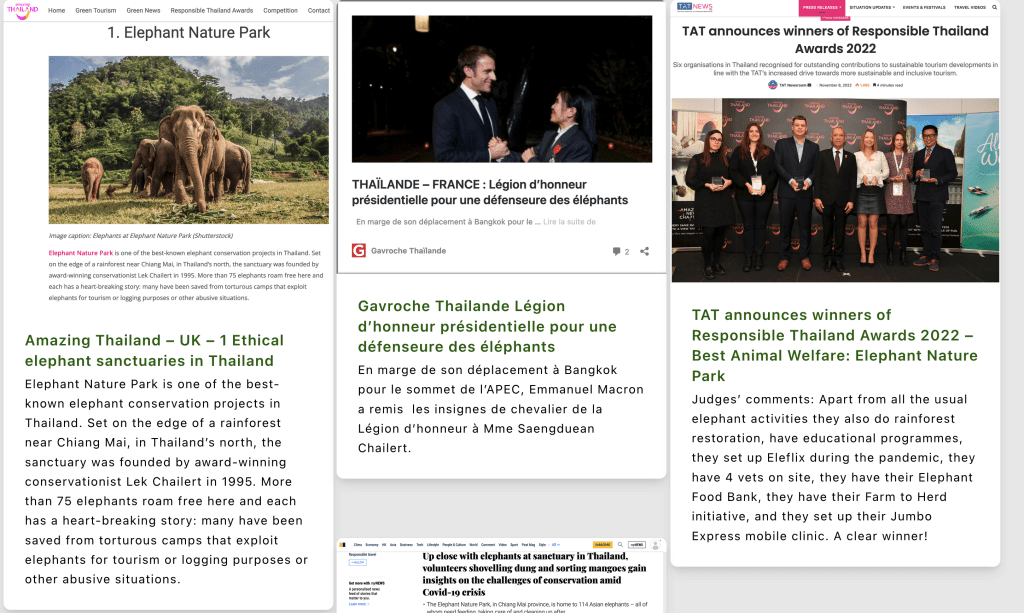### Screenshot from Desktop or Laptop Displaying a Travel Website

At the top of the screenshot, there is a prominent pink header that appears to contain the word "Thailand." Below the header, there are several navigation links including "Home," "Green Tours," "Green News," "Responsible Thailand Awards," "Competitions," and "Contact."

The main content is divided into three primary articles and a fourth partially visible one at the bottom. 

1. **Left Article: "Elephant Nature Park"**
   - **Image**: Shows several elephants in a lush, green park with dense foliage in the background.
   - **Title**: "Amazing Thailand UK, One Ethical Elephant Sanctuaries, the Number 1 Ethical Elephant Sanctuaries in Thailand."
   - **Description**: Details the Elephant Nature Park, a renowned elephant conservation project located on the edge of a rainforest near Chiang Mai in northern Thailand. Founded in 1995 by award-winning conservator Lek Chalert, the sanctuary is home to over 75 elephants, many of which have been rescued from abusive situations in tourism and logging camps.

2. **Middle Article**: 
   - **Image**: Features an actor and an Asian woman, seemingly greeting each other and clasping hands.
   - **Text**: The article appears to be written in French, making it difficult to decipher for non-French readers.

3. **Right Article: "TAT Announces Winners of Responsible Thailand Awards 2022"**
   - **Image**: Depicts seven individuals holding awards.
   - **Description**: Highlights the judges' comments on the award winners. Aside from traditional elephant activities, they contribute to rainforest restoration, have educational programs, set up Elefix during the pandemic, employ four on-site vets, run an elephant food bank, initiate farm-to-hood projects, and established the Jumbo Express mobile clinic. 

This detailed caption aims to provide a comprehensive overview of the screenshot, making it easier to understand the context and content of the displayed articles.